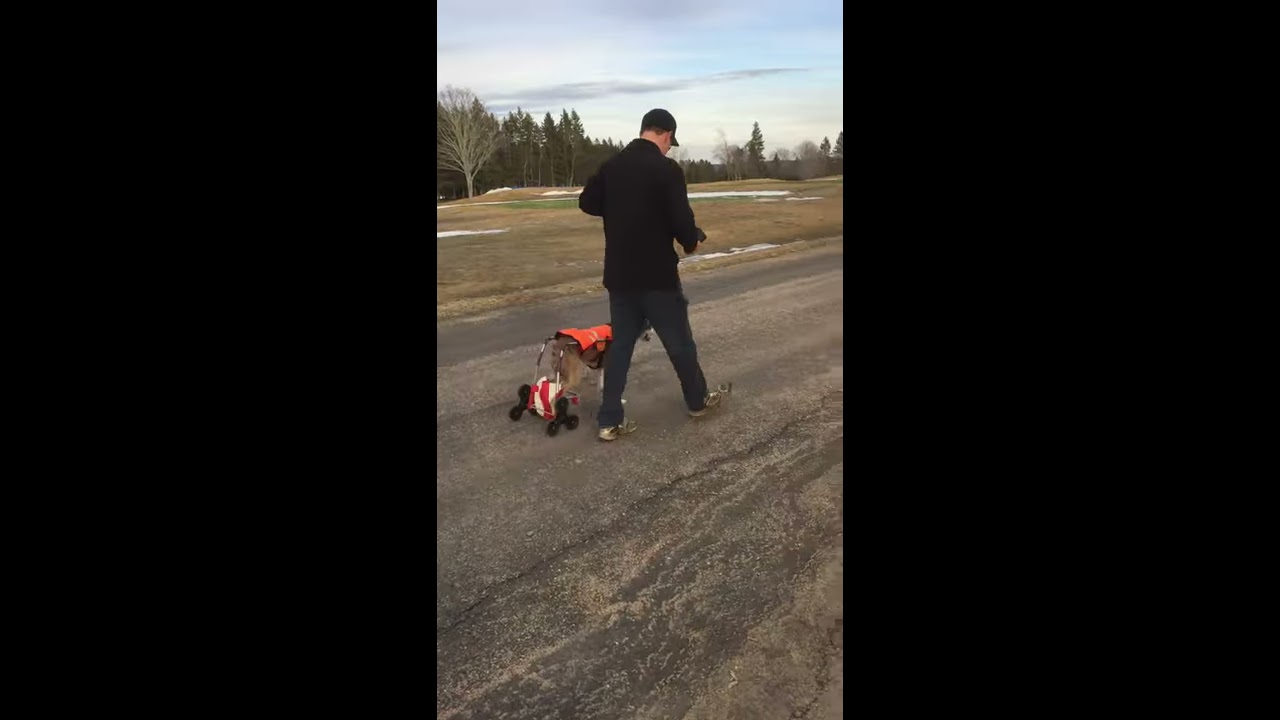An image divided into three vertical sections, with the outer sections entirely black, and the middle section showcasing a vivid outdoor scene. The main focus is a man and his dog, walking along a light-colored, slightly grainy asphalt road that has patches of sand or dirt. The man, facing away at a three-quarter angle to the viewer, wears a black cap, a black long-sleeved shirt or jacket, dark blue pants, and brown shoes. He appears to be Caucasian with brown hair and is stepping forward with his right foot. Beside him on his left, the dog, clad in an orange vest, is utilizing a wheeled apparatus to support its hind legs, indicating it might be handicapped. The scene is set on a sunny day with blue skies dotted with white clouds. Adjacent to the road is a large, empty field covered with dry, brown grass interspersed with patches of snow. Further in the distance, a row of trees marks the horizon.